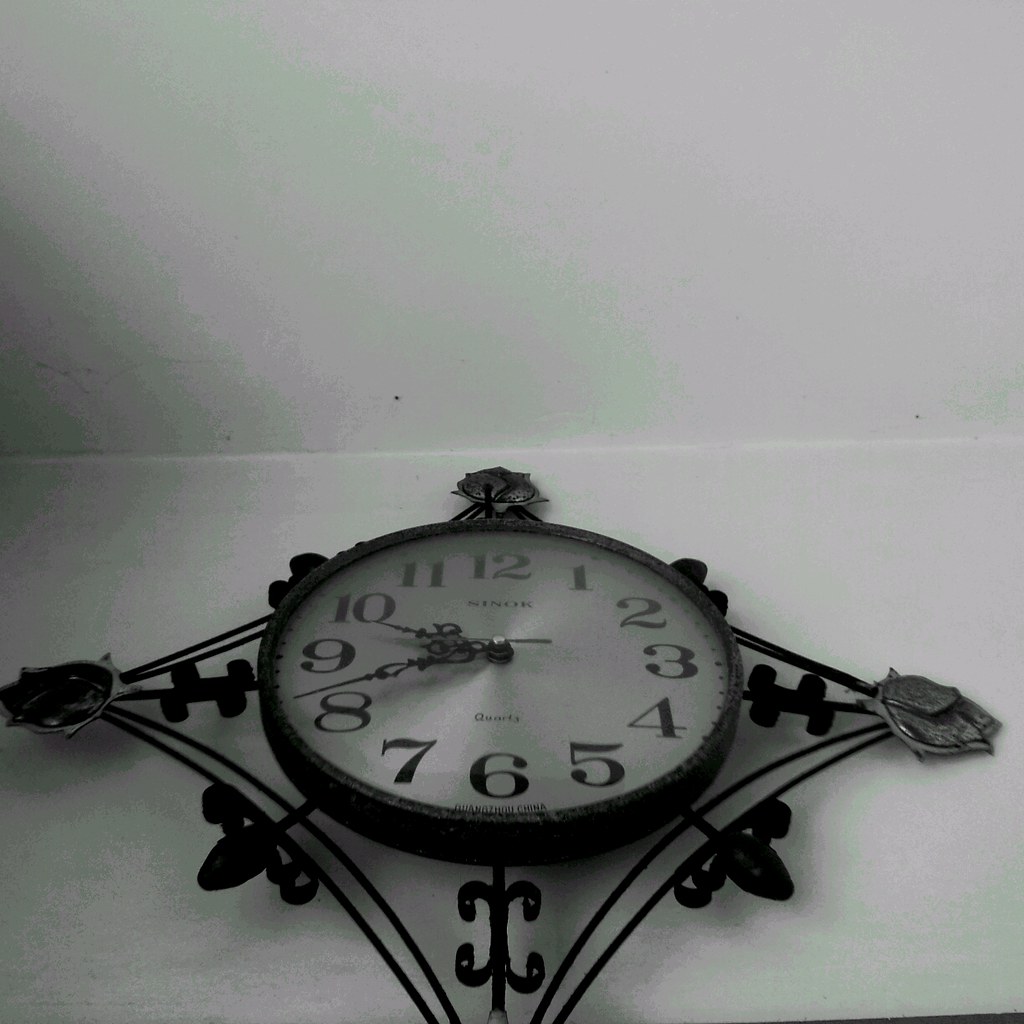In this image, you see an elaborate wall clock positioned on a bright white wall with a matching white ceiling, viewed slightly from below. The clock itself is circular, featuring a white face with bold black numbers from 1 to 12, and ornate, intricately detailed black hands. The clock is set in a black, glossy metal frame designed to mimic wrought iron, forming a striking diamond shape surrounding the clock. The decorative frame includes fleurs-de-lis and floral elements at the tips of the diamond shape. This intricate metalwork, resembling double-wired black spokes, connects the clock to the wall, enhancing its ornate appearance. The visible time on the clock is roughly 9:42.